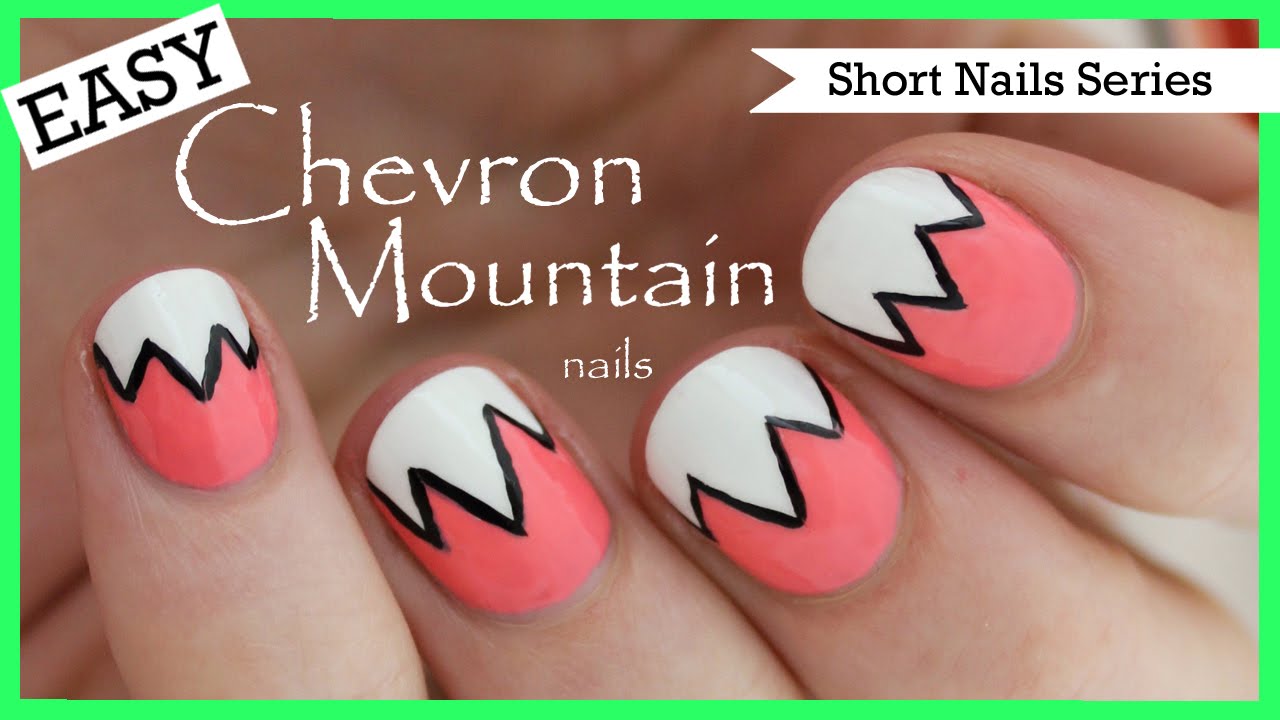The close-up image showcases four well-manicured fingers, each adorned with a stylish chevron mountain design. The nails are part of a tutorial for a "Short Nails Series" and are painted with a peach-pink base at the cuticles, transitioning into a black zigzag line across the middle, and topped with a white tip. Enhancing the visual appeal, the photo is framed by a neon green border with white text that reads "Easy Chevron Mountain Nails." It's evident from the image and accompanying details, including the logo visible on the thumbnail, that this is part of a YouTube series. The image also promotes Beadaholique.com for beading supplies.